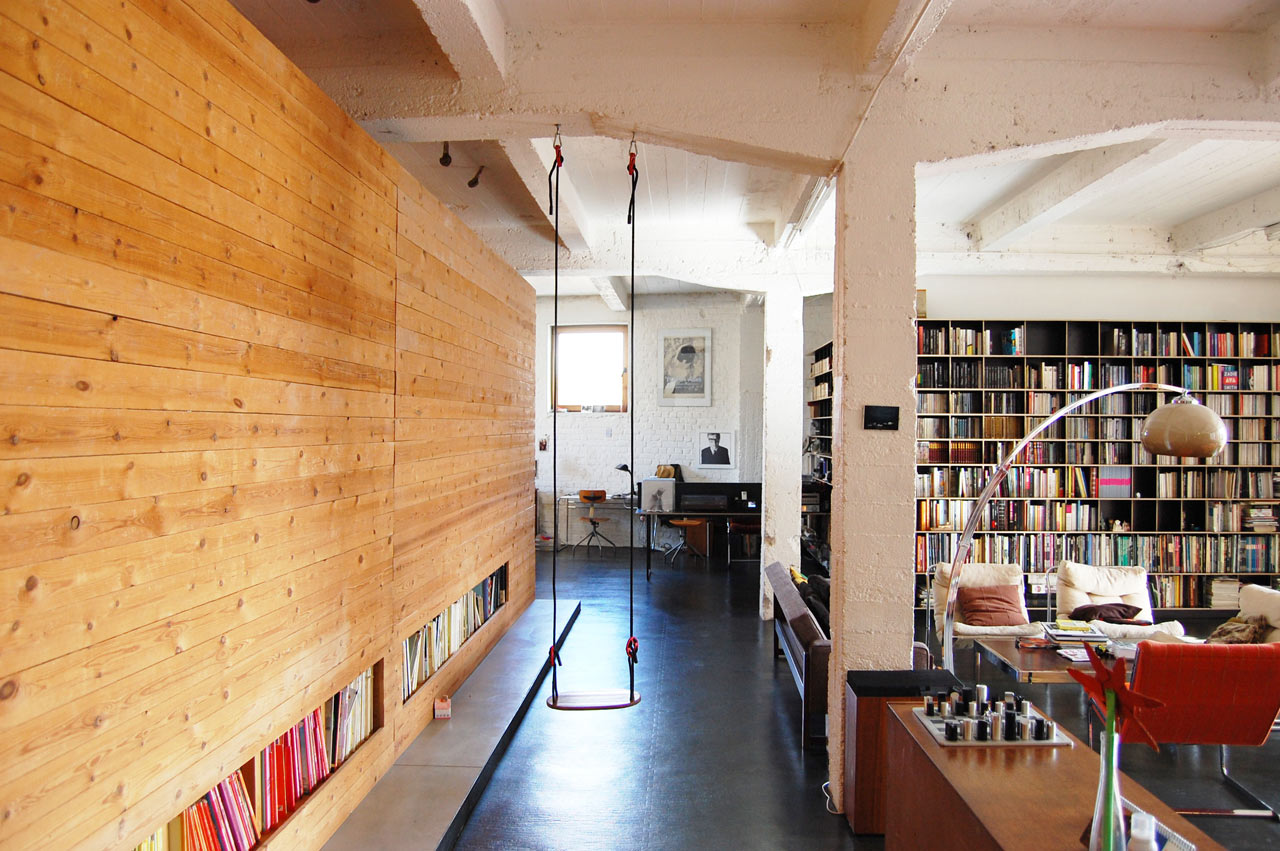This interior photo captures a potential library or study hall, characterized by a blend of modern and rustic elements. On the left, a wall adorned with vertically aligned pine boards extends towards the center. Below the wall, various openings reveal a multitude of books. Dominating the scene, a swing with a beige seat and red ribbons hangs from the ceiling beams in the hallway.

To the right, a series of wooden tables, including one with a checkerboard, are neatly arranged. An arc lamp illuminates a table surrounded by chairs with brown pillows, suggesting spaces for both study and casual conversation. A modern chess set and a vase with a single-stemmed flower are also visible, adding detail to the ambiance.

Further in the distance, large bookshelves brimming with books stretch along the back and left side of the room. The ceiling, supported by concrete girders, hints at a substantial structure possibly part of a college campus or an office building. The floor is shiny linoleum, adding a touch of practicality to this multifaceted space, which also features desks and a picture on the far wall, enhancing the scholarly atmosphere.